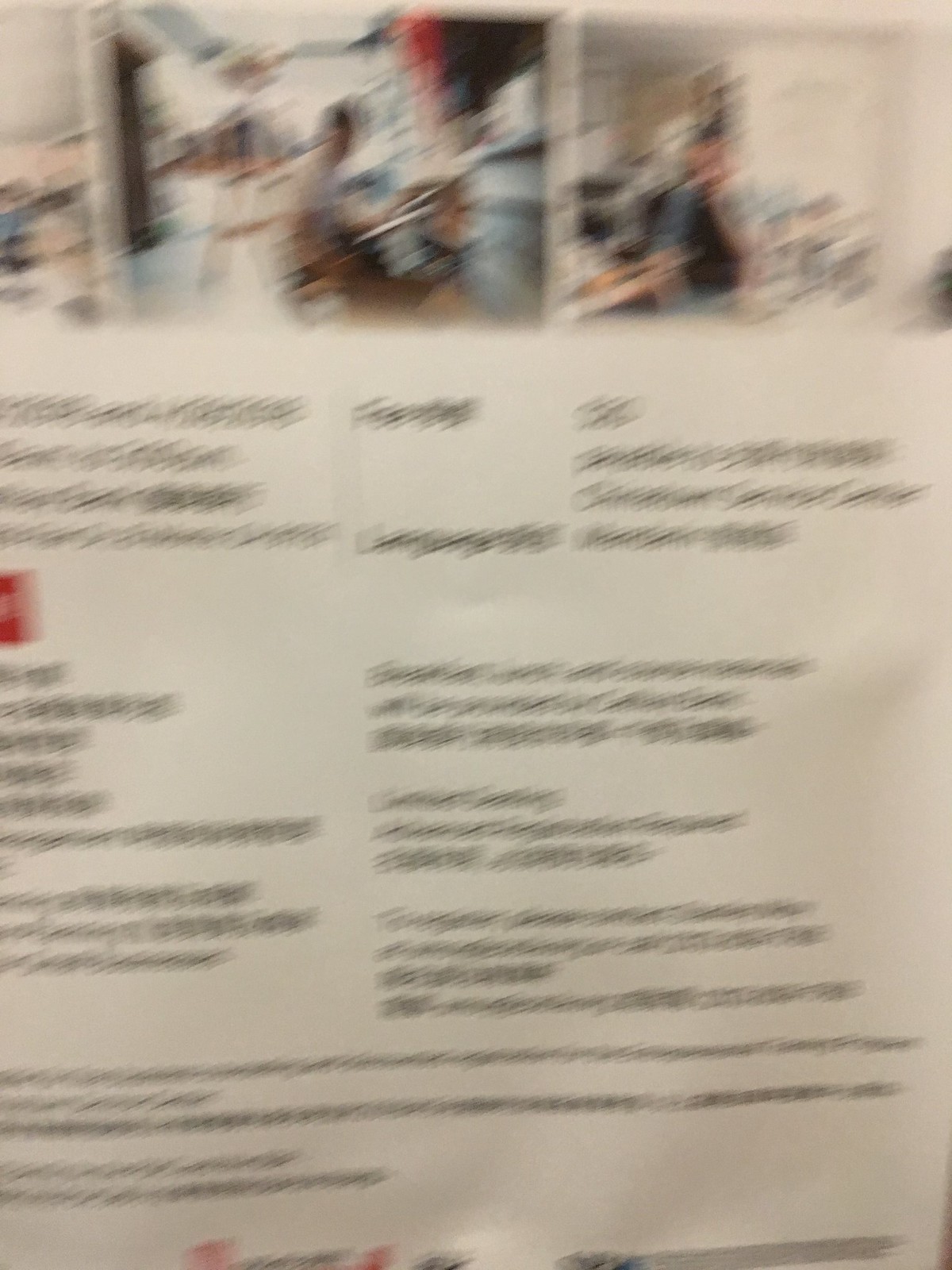The photograph is a blurry close-up of a piece of white paper, possibly a poster or a printed document. At the top of the paper, there are several blurry images. The picture on the top left appears to depict someone sitting down, though the details are indistinct. The image on the top right is unidentifiable due to the blur. Below these images, there are blocks of black text, which might be intended to describe or provide context for the images above. The text is printed on standard white paper.